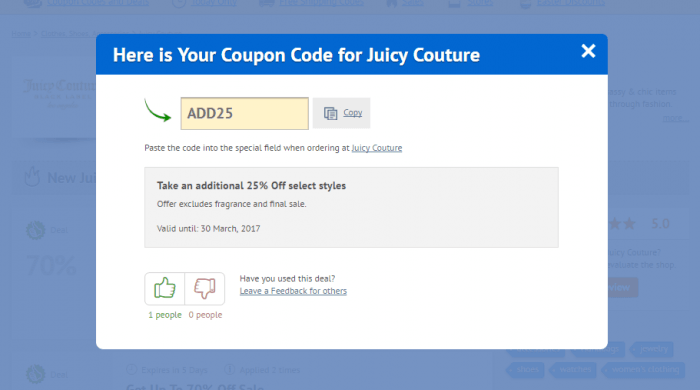The screenshot captures a pop-up menu on a website, which creates a lilac-colored overlay on the rest of the page, rendering the background unreadable and obscured. The pop-up is centered on the screen and is predominantly white with a blue bar at the top. In the blue bar, written in white font, is the text, "Here is your coupon code for Juicy Couture," along with a small white 'X' in the top right corner for closing the menu. Below this blue bar, in the white section of the pop-up, there is a beige rectangle containing the text "ADD25" in black font, with a red arrow pointing to it for emphasis. Adjacent to the beige rectangle is a small gray icon of two overlapping pieces of paper, next to which is the word "Copy" in blue font. Further down the pop-up, there's an instructional message that reads, "Paste the code into the special field when ordering at Juicy Couture." At the bottom of the pop-up, inside a gray rectangle, there's an additional offer statement, "Take an additional 25% off select styles."